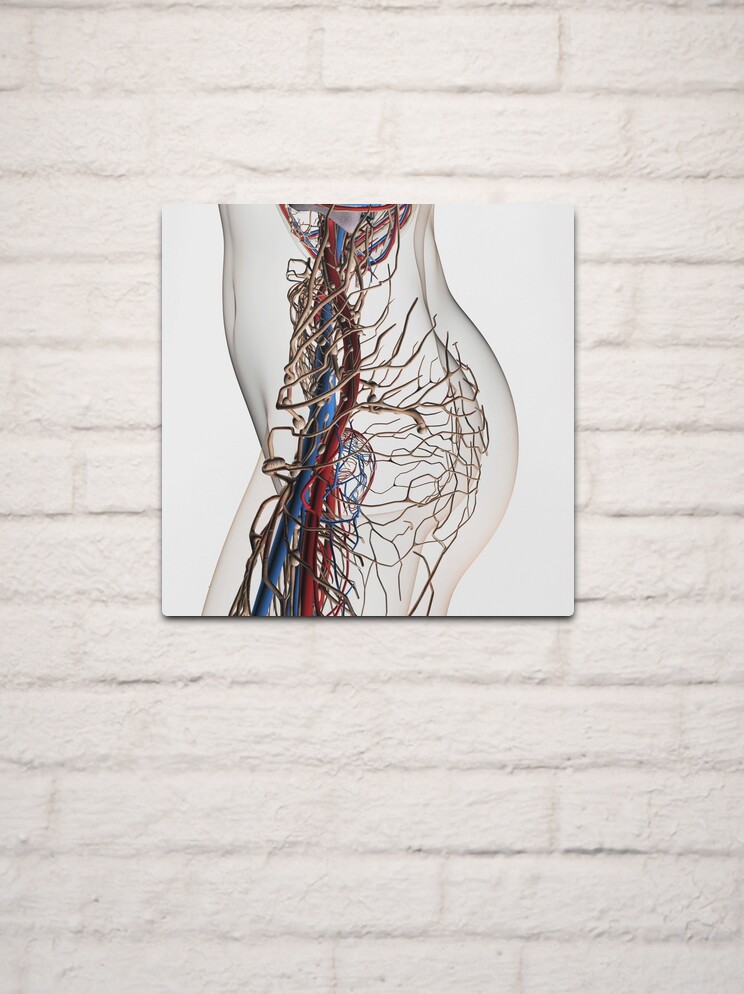This image features a square piece of art with rounded corners, mounted on a white-painted brick wall. The artwork, printed on what appears to be an aluminum or metal sheet, portrays an anatomical side profile of a woman's lower torso, spanning from the ribcage to the mid-thigh, all against a stark white background. The profile is outlined in gray and showcases a detailed depiction of the circulatory system with thick red arteries and blue veins running parallel through the body's hip area. Additionally, there are smaller tan-colored veins and possibly a network of brownish elements that could represent the nervous system. The intricate network resembles tree roots, vividly illustrating the complex vascular structure within the semi-transparent, gray-toned silhouette of the body.